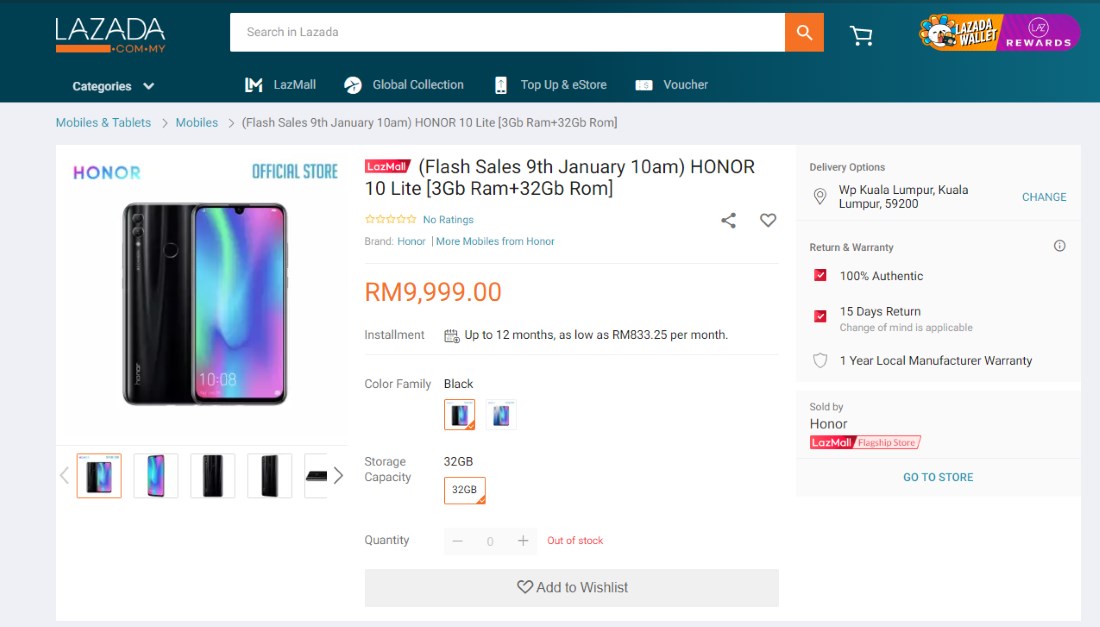**Detailed Description:**

**Lazada Mobile App Screenshot Overview**

- **Top Left Section:**
  - A cell phone depicted on the left side of the screenshot.
  - A dark blue bezel at the top displays the name "LAZADA" in white text.
  - Right beneath, an orange rectangle is followed by ".com.my" in the same color.

- **Search and Navigation Bar:**
  - A white search bar with grey text that says "search LAZADA."
  - An orange square at the end of the search bar featuring a white magnifying glass icon.
  - A white shopping cart icon located outside of the search bar.
  - An oval button on the far right side showing a white bear-like figure holding a camera, surrounded by alternating orange and blue balloon-like elements. Beside the icon, it says "LAZADA wallet" with an orange background, and the section looks like a pill split into a purple half with a white circle labeled "LAZ" and "rewards" in bold white text.

- **Tabs and Icons:**
  - Multiple tabs grouped in the blue area:
    - "Categories" in bold white with a downward arrow.
    - "LM" in bold white beside "LAZMALL" in regular white.
    - A white circle with a plane icon labeled "global collection."
    - An icon resembling a cell phone with the text "top up and e-store."
    - A rectangle with the text "voucher."

- **Product Listing:**
  - Tabs indicating product categories:
    - A cyan blue tab labeled "mobiles and tablets."
    - Mobiles underlined with cyan blue, followed by a grey arrow.
    - A grey arrow pointing to "flash sale is 9th January 10am" in parenthesis (indicating a special offer date).
  - Brand info:
    - "HONOR" in all caps and "10LIGHT" in brackets, denoting a model with "3G RAM + 32GB ROM" in smaller text.
    - A visual of the cell phone's back (black) and a colorful front display with bands of blue, green, pink, purple, and hot pink. "1008" is visible at the bottom left.
  - Pricing and Store Info:
    - Price shown in orange "RM 9999.00" (indicating a different currency, likely Malaysian Ringgit).
    - "Official store" at the top right, "HONOR" on the left with multi-colored letters transitioning from purple and pink to blue and teal.
  - Additional product specifics:
    - A red rectangle labeled "Laz Mall" with white text and a note about the flash sale timing in parenthesis.
  
- **Product Ratings:**
  - No ratings are indicated by unselected stars and the phrase "no ratings" in italicized blue.
  - "Brand" in black text with "HONOR" listed underneath.
  - Suggestion to explore more mobiles from "HONOR" in blue.

- **Purchase and Payment Options:**
  - Installment plans detailed in grey text:
    - Up to 12 months duration, as low as RM 833.25 per month.
  - Product color family "black" is selected (highlighted by an orange border).
  - Storage capacity options listed:
    - 32GB is selected but out of stock (highlighted in orange, with "out of stock" in red).
  
- **Additional Details:**
  - A dark grey rectangle with black text that says "add to wish list" and features a heart icon.
  - Delivery options:
    - "WP KUALA Lampur 59200" indicated with a location pin.
  - Authenticity and return policy details:
    - A red square stating "100% authentic."
    - Another red square stating "15 days return" with a note "change of mind is acceptable."
    - A grey shield outline mentioning "one year local manufacturer warranty."

This comprehensive description captures all the essential elements visible on the Lazada app screenshot, elucidating colors, text, icons, and nuanced details to provide a clear understanding to the reader.